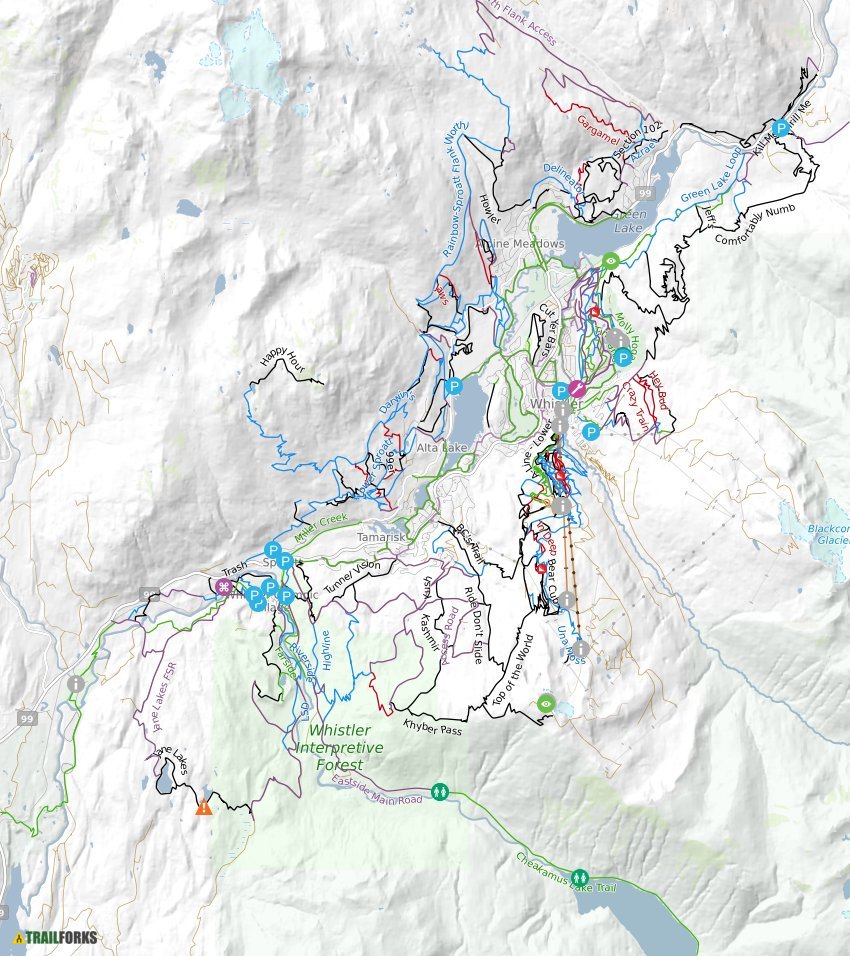This image showcases a detailed, wrinkled paper map predominantly with a white background, filled with various marked trails in an assortment of colors: green, black, purple, blue, and red. The map highlights a forested area, likely intended for hiking, aptly labeled "Whistler in Interpeth Forest." The map features numerous points of interest, including bodies of water like Green Lake, Alta Lake, and Miller Creek, and locations such as Tunnel Vision, Camber Pass, Top of the World, Ride Don't Slide, Glacier, Molly Hood, Crazy Train, and Haybird.

Key symbols are dispersed throughout the map: green circles with human figures, blue circles marked with the letter "P" for parking, gray circles with the letter "I" for information, and a purple circle with a wrench indicating repair points. There’s also an orange triangle with an exclamation point for cautionary notices. Contour lines trace the elevation changes across the terrain, denoting peaks and valleys. In the bottom left corner, the map credits "Trailforks" with its creation, indicated by black and green text alongside a distinctive yellow triangle with a black symbol.